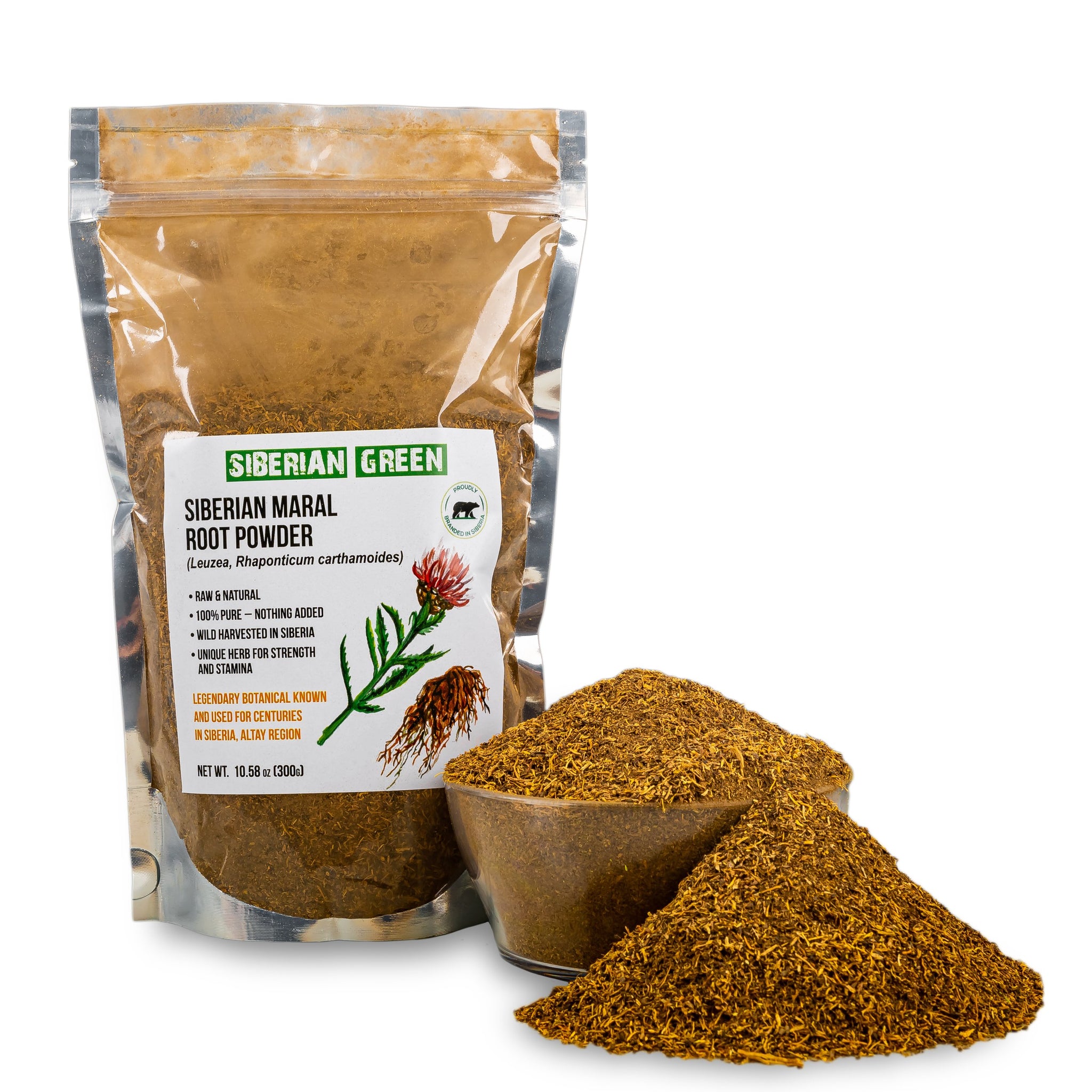This image showcases a transparent plastic bag with a zip-top seal and a tear-open feature. The label prominently reads "Siberian Green" in white font against a green background, and "Siberian Marl Root Powder" in black text. Beneath this, there is some unreadable font, and an illustration of a green plant with pink blooms. The powder within the bag is visible and appears brown, resembling finely ground dirt or leaves. To the right of the bag, a bowl contains more of this brown powder, with a small pile of the same substance on the ground beside it. The entire scene is set against a white background, reinforcing the focus on the product. This is a promotional image emphasizing the natural, 100% pure quality of the Siberian Marl Root Powder, a historically significant herb known for its strength and stamina benefits, wild-harvested in Siberia's Althae region.